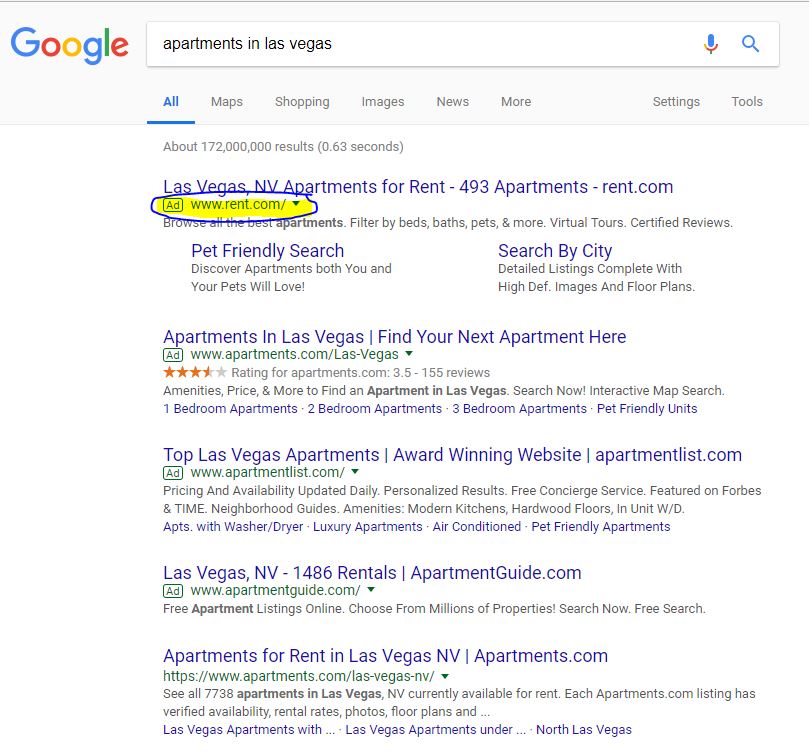In the image, someone has performed a Google search for "apartments in Las Vegas" and highlighted the search results. The top result, outlined with a blue circle, is titled "Las Vegas, Nevada apartments for rent" from the site 493apartments-rent.com. This listing invites users to "browse all the best apartments, filtered by bedrooms, bathrooms, pets, and more." Below it, options in blue text include "pet-friendly search" and "search by city."

The second result is from www.apartments.com, urging prospective renters to "Find your next apartment here." This listing details various amenities such as pricing, availability, one-bedroom, two-bedroom, three-bedroom apartments, and pet-friendly units.

Following that, there's an entry from apartmentlist.com, branding itself as an award-winning website with "top Las Vegas apartments." It boasts features like daily updated pricing and availability, personalized results, free concierge service, modern kitchens, hardwood floors, in-unit washer-dryer, luxury amenities, air conditioning, and pet-friendly options.

The fourth result is from apartmentguide.com, listing "1,486 rentals in Las Vegas, Nevada." It offers free online apartment listings and encourages users to "choose from millions of properties" and "search now for free."

Finally, the last listing is from apartments.com, co7.com, indicating "7,738 apartments in Las Vegas, Nevada, currently available for rent." This site includes verified availability, rental rates, photos, floor plans, and more. The caption concludes by noting this comprehensive Google search for apartments in Las Vegas.